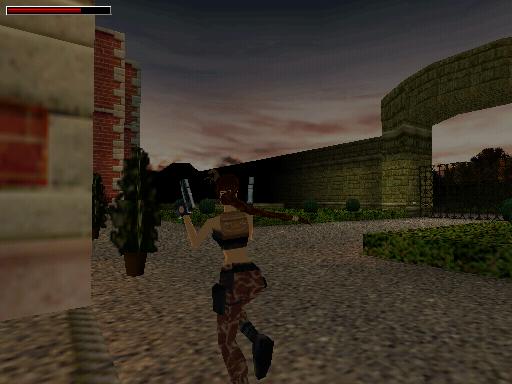The image is a screenshot from a video game, possibly a Tomb Raider installment, characterized by its dark, nighttime setting with a slightly lighter horizon. Dominating the scene is a woman with a long, reddish-brown ponytail, dressed in a brown tank top and brown camouflage pants. She is positioned in the center, facing away from the viewer, running along a textured cobblestone street that stretches and curves to the right. In her hands, she clutches two pistols, with holsters on her hips, and one of her black shoes is visible at the bottom of the image. The environment includes short hedges around her, a large gate ahead, and a prominent brick wall extending from a brick arch to the right. A rectangular status bar in the upper left shows a three-quarters filled red bar against a black background. The setting appears to be outside a mansion with cobblestone roadways, surrounded by grass and gray brick structures.